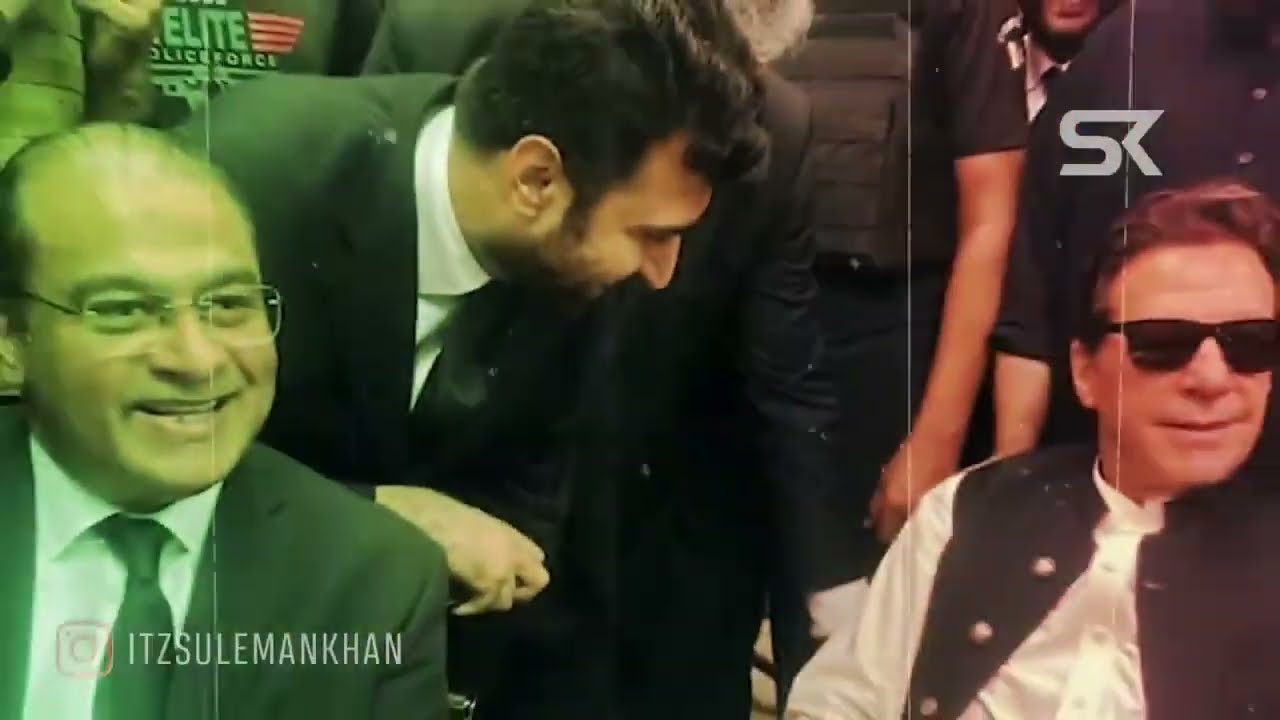The image captures a lively scene, likely set at a crowded event such as a sporting event or a press conference, characterized by its grainy, Polaroid-like effect. The foreground is dominated by three men, all smiling, forming the central focus. 

On the left, a man around 40 years old or older, with a bald top head and wearing clear-framed glasses, sports a toothy grin. He is dressed in a black suit with a black tie. In the middle, a man of Indian descent, also clad in a black suit, is crouching down, engaging directly with the man on the right, sharing a toothy smile. Finally, on the right, a white-skinned man with dark hair and wearing black sunglasses sits comfortably, displaying a smirk. He is dressed in a black button-up vest over a sheer, satin-like long-sleeve button-up shirt. 

The setting is well-lit with natural light, contributing to the clear and bright quality of the image despite its film-like texture. Visible in the bottom corners are watermarks and the Instagram handle "ITZSULEMANKHAN." In the background, only legs and torsos are visible, indicating a larger crowd beyond the frame.